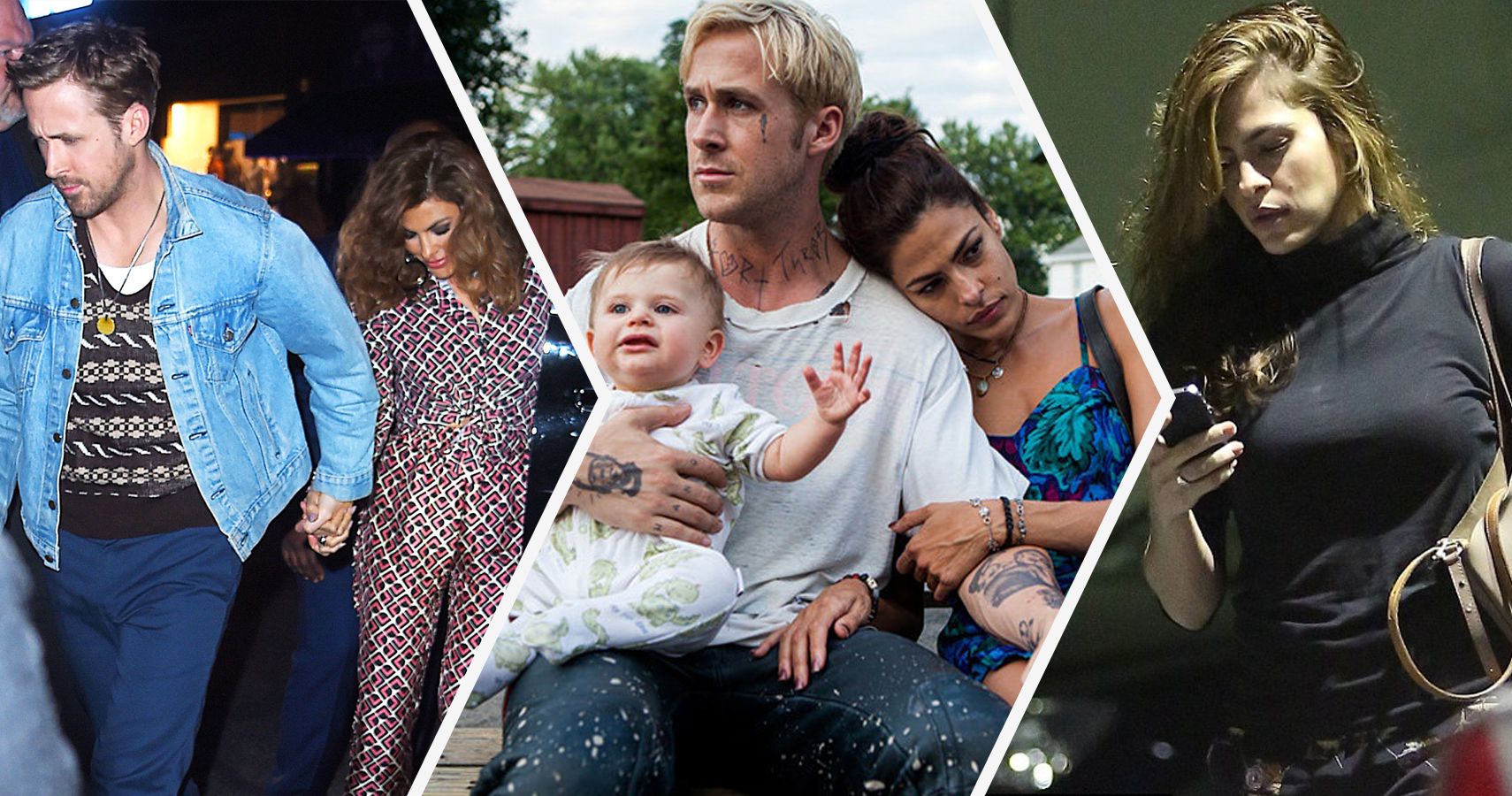The image is a three-photo collage featuring Ryan Gosling and Eva Mendes. The first picture on the left shows Ryan Gosling holding hands with Eva Mendes. He is dressed in a jean jacket over a striped sweater vest, wearing blue pants. He has brown hair and a beard. Eva Mendes, walking slightly behind him and likely trying to avoid paparazzi, wears a geometric-patterned jumpsuit in shades of red, black, white, and possibly yellow. The middle image portrays Ryan Gosling with bleached blonde hair, a white torn t-shirt, and sporadically spattered jeans. He has tattoos on his neck, hands, and forearms, and is holding a baby in a white onesie on his knee. Eva Mendes, with her hair tied up in a bun, is resting her head on his shoulder, wearing a blue and green tank top with magenta accents. The rightmost image focuses on Eva Mendes, now with long reddish-blonde hair swept to the left. She is dressed in a plain black turtleneck and carries a purse over her shoulder, engrossed in her cell phone while walking. Each photograph, separated by white arrow-like divisions, captures different moments of the couple, highlighting their casual yet intimate interactions.